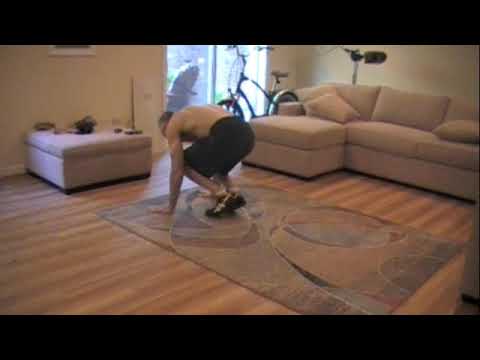The image depicts a shirtless, older, fit, and skinny man performing exercises, such as a push-up or burpee, in his well-lit living room. He is crouched down with his hands on a rectangular carpet, wearing black shorts and running shoes. The living room features a central, square carpet placed on a hardwood floor, bordered by a cream-colored sectional sofa with a corner unit and matching cream-colored throw pillows. In front of the man is a large beige ottoman, and behind him, the room is brightened by natural light pouring through a wide sliding glass door. Leaning against the door is a bicycle. The walls of the room are off-white, and there is possibly a tripod or lamp behind the couch. The overall scene suggests a bright and clear daytime setting.